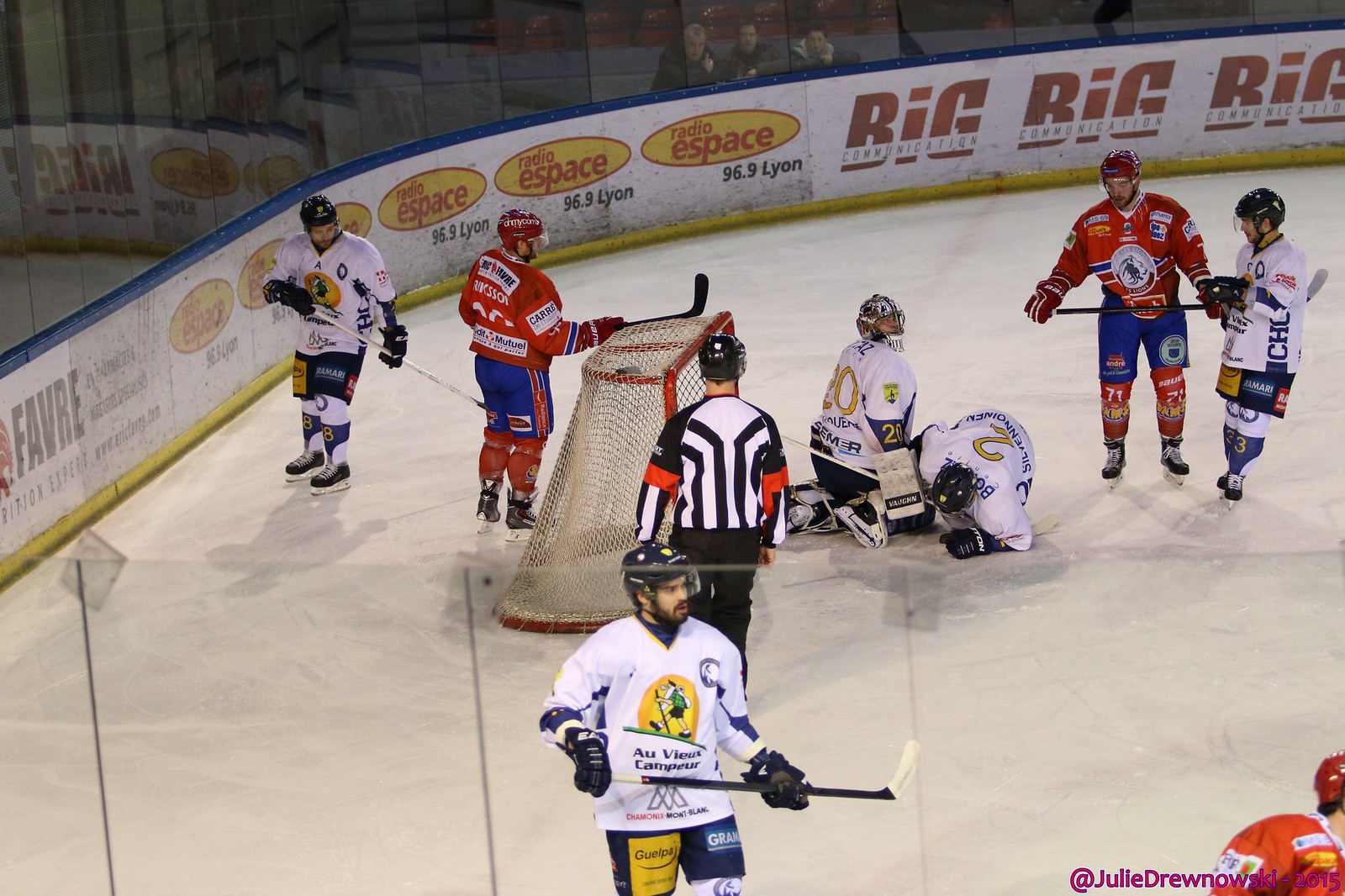The image is a detailed photograph of a hockey game taken from the stands on the left side of the ice rink. The main focus is on the goal on the left side, which has red poles and a white net. The goalie, dressed in a white jersey, black helmet, and blue shorts, appears to have just captured the puck. Surrounding the goalie are four players in the same white uniform and three players in red jerseys, blue shorts, and red helmets. The referee stands directly in front of the net with his back turned to the viewer. Behind the glass wall that encircles the rink, there are visible advertisements and fans closely watching the game. The stands in the background are red, indicating that the photo was taken in a hockey arena. Additionally, there is prominent text that reads "96-something AM" visible in the background. The players’ positions vary, with some standing around the goal area and others scattered across the ice. The image captures a dynamic moment with all the players focused on the goalie, who seems to be either on the ground or in a low stance after making the save. The lighting of the arena doesn’t give clear cues on whether the game is taking place during the day or night.